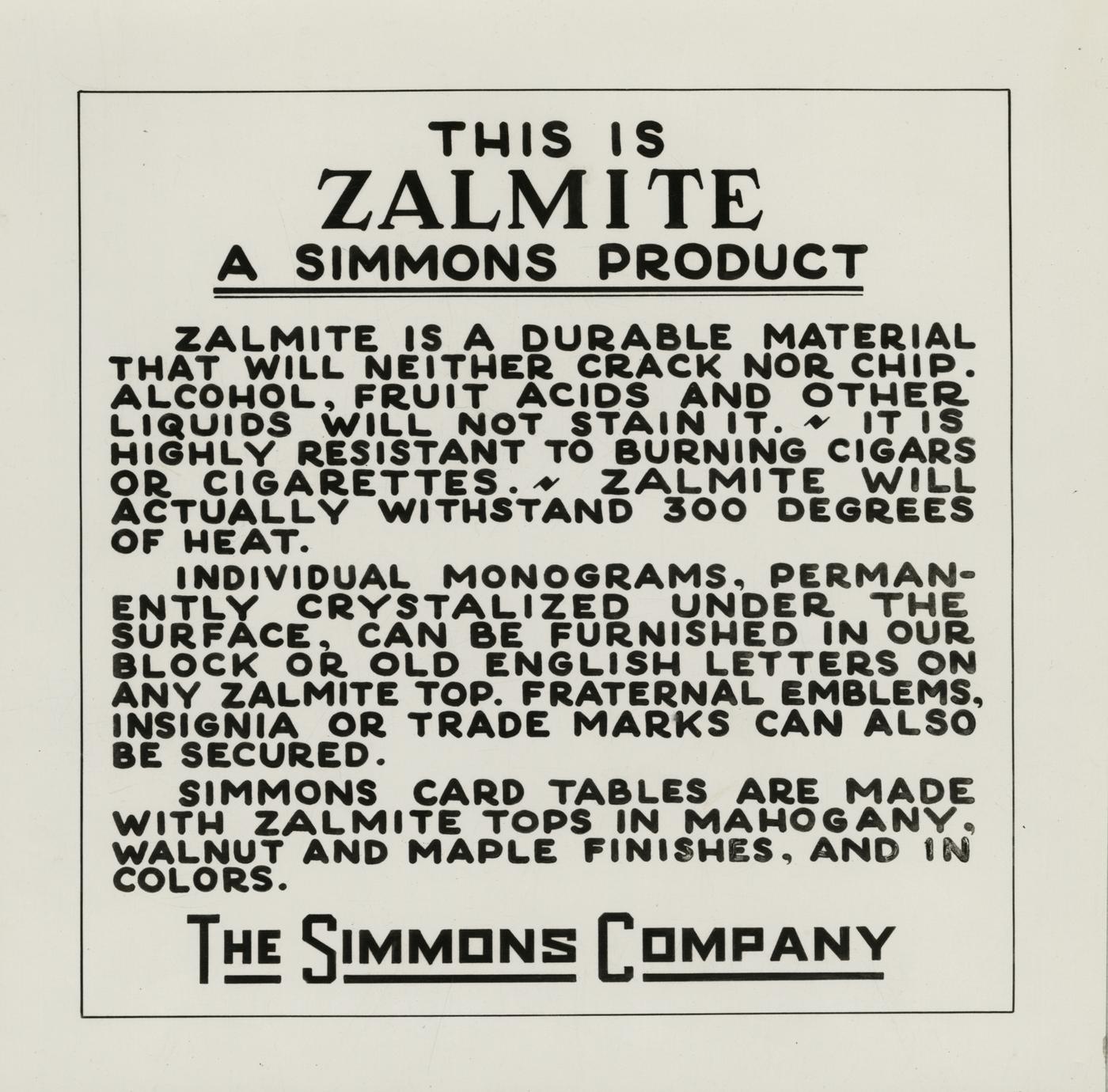This image is an old advertisement for Zalmite, a durable material produced by the Simmons Company. The advertisement is set against an off-white background with a thin black line border around the text. At the top, in large black capital letters, it states: "This is Zalmite, a Simmons product," which is underlined with a double line. The text describes Zalmite in detail, highlighting its durability and resistance to damage. Zalmite neither cracks nor chips, and it is impervious to stains from alcohol, fruit acids, and other liquids. It can withstand heat up to 300 degrees Fahrenheit, making it highly resistant to burning cigars or cigarettes. The material can also be customized with permanent monograms, available in block or old English letters, as well as fraternal emblems, insignia, or trademarks. The advertisement further mentions that Simmons card tables are made with Zalmite tops and are available in mahogany, walnut, and maple finishes, along with various colors. At the very bottom, it prominently features "The Simmons Company," with underlines beneath each word.